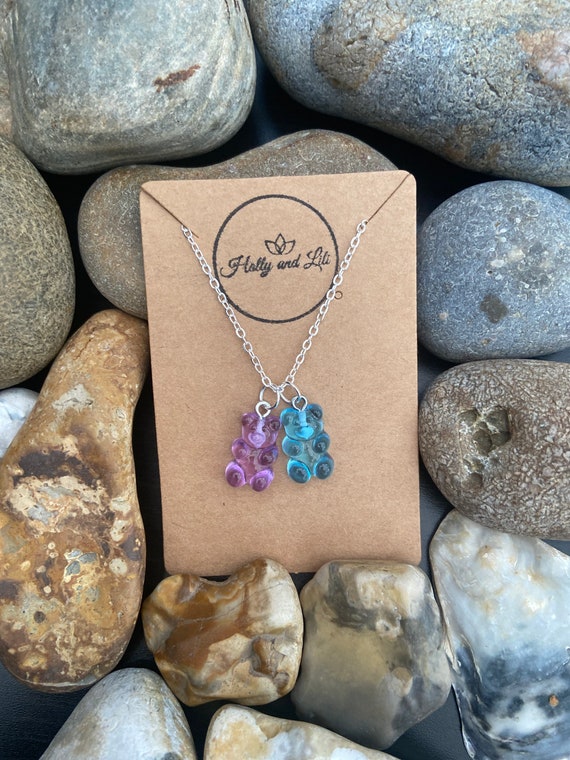This photograph features an intricately crafted necklace designed by Holly and Lily and serves as an advertisement. The necklace, composed of a delicate silver chain, showcases two charming, transparent gummy bear pendants - one in a purple hue and the other in aqua blue. These pendants are carefully suspended from a piece of rectangular brown craft paper, which has slits to hold the chain in place. The backdrop consists of an array of smooth, polished river rocks in varying shades of gray, brown, tan, and white, providing a natural and earthy setting that contrasts beautifully with the vibrant colors of the gummy bear charms. At the top middle of the craft paper, a circular logo with a flower motif bears the brand name "Holly and Lily." The harmonious arrangement of elements in the image highlights the playful elegance of the necklace, making it an eye-catching promotional display.